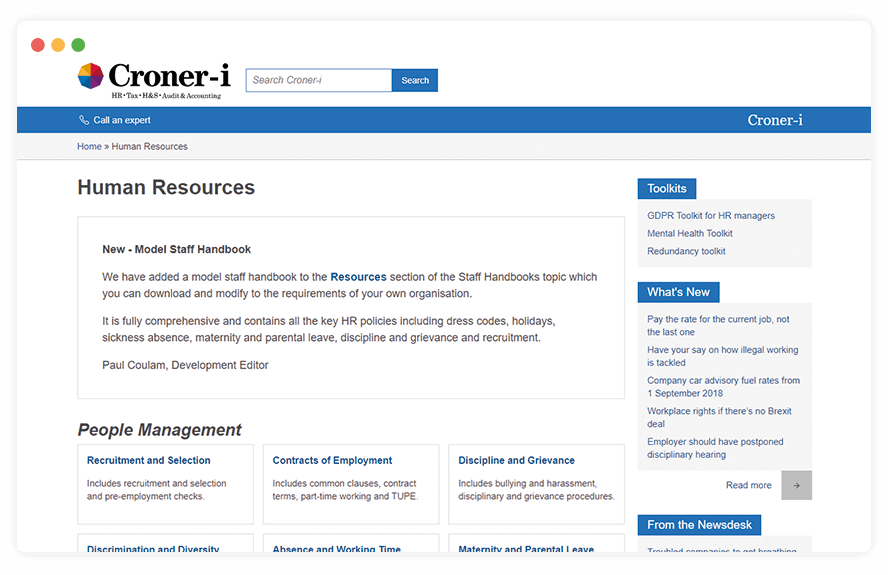**Detailed Caption:**

This screenshot depicts the homepage of Croner-I, a platform specializing in HR, Tax, Health & Safety, Audit, and Accounting. At the top of the page, the Croner-I logo is prominently displayed. Below it, the website offers a range of navigational options including Home, Human Resources, and others. The central focus is on Human Resources, showcasing a New Model Staff Handbook added to the Resources section within the Staff Handbooks topic. This comprehensive handbook is customizable to meet the specific requirements of various organizations and includes essential HR policies covering dress codes, holidays, sickness, absence, maternity and paternal leave, discipline and grievance procedures, and recruitment guidelines.

Additionally, the page highlights key sections like People Management and Recruitment and Selection, which detail the recruitment process and pre-employment checks. The Contracts of Employment segment outlines common clauses, contract terms, part-time working, and TUPE regulations. The Discipline and Grievance section addresses bullying and harassment, disciplinary and grievance procedures, discrimination and diversity, along with policies on absence and working time, and maternity and parental leave.

To the right side of the screenshot, a Toolkits section lists valuable resources including the GDPR Toolkit for HR Managers, Mental Health Toolkit, and Redundancy Toolkit. The What's New section features updates such as "Pay the Rate for the Current Job, Not the Last One," "Have Your Say on How Illegal Working is Tackled," "Company Car Advisory Fuel Rates from 1 September 2018," "Workplace Rights if there is no Brexit deal," and an article titled "Employer should have postponed disciplinary hearing." There is also a prompt to "Read more from the News Desk."